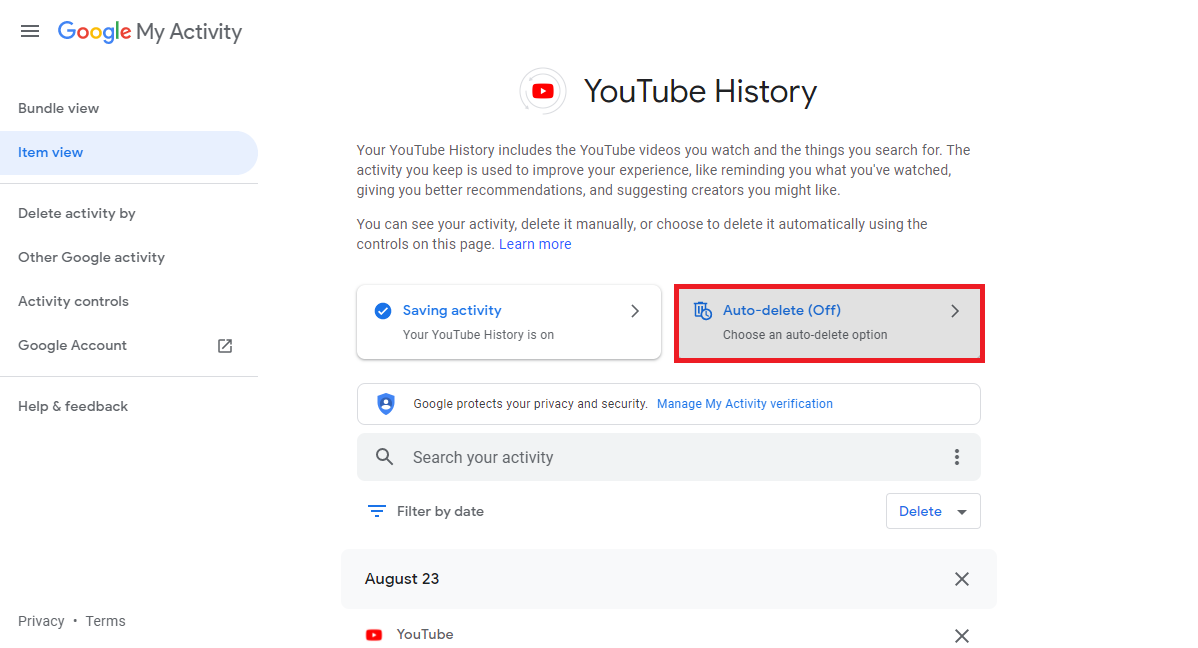This image is a detailed screenshot of someone's Google My Activity dashboard, focusing on their YouTube history. In the top left corner, the interface is labeled "Google My Activity," with a variety of tabs displayed horizontally. These tabs include "Bundle View," "Item View" (currently highlighted in blue, indicating the active tab), "Delete activity by," "Other Google activity," "Activity controls," "Google account," and "Help and feedback." In the bottom left corner, there is a "Privacy and terms" link.

The right side of the screenshot centers on the YouTube history section. Prominently, there is a button labeled "Saving activity," with the status "Your YouTube history is on," accompanied by a check mark. To its right, an "Auto-delete" option is visible and is currently turned off, highlighted in red. Below these controls, Google emphasizes its commitment to privacy and offers options like "Google Protects Your Privacy" and "Manage My Activity Verification."

A magnifying glass icon sits adjacent to a search box, allowing the user to filter activities by dates. Next to this, there is a "Delete" button. The activity recorded on this date is marked as August 23rd. Following this date label, an entry lists "YouTube" alongside its recognizable icon, with an "X" button right-aligned, providing an option to delete specific entries.